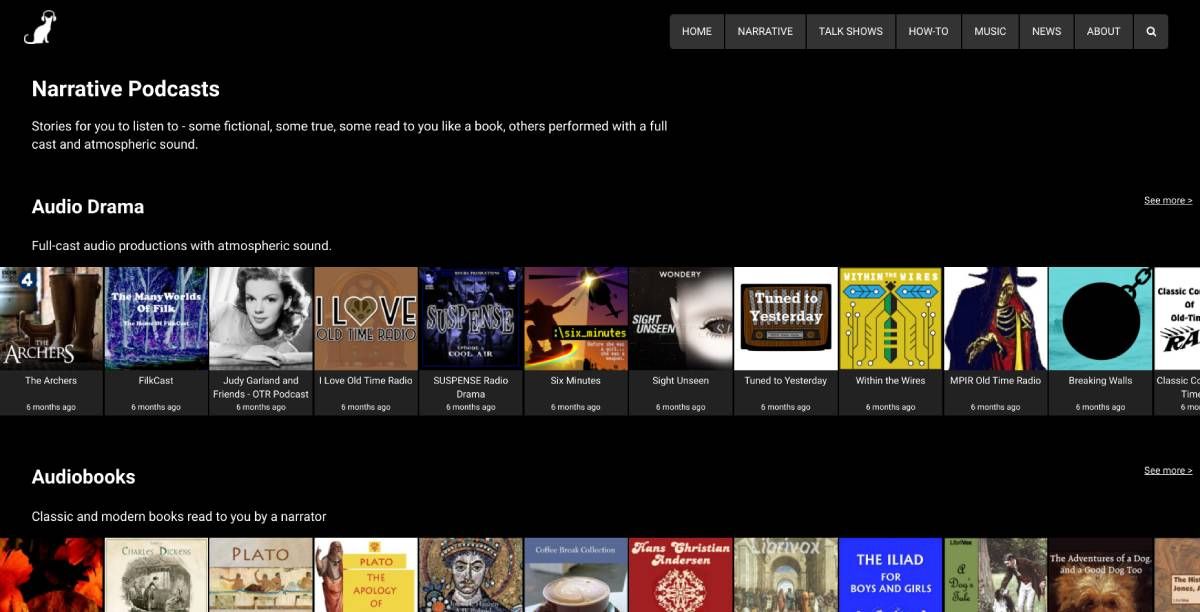The website features a sleek, primarily black design. In the top left corner, there is a distinctive white logo resembling a dog sitting upright with its two front paws on the ground. On the far right side, the navigation menu is displayed in gray squares with white font, containing options labeled: Home, Narrative, Talk Shows, How-To, Music, News, About, and a magnifying glass icon for search functionality.

On the left side, prominently displayed in bold font, is the title "Narrative Podcasts." Below it, in unbolded font, is the subtitle: "Stories for you to listen to, some fictional, some true, some read to you like a book, others performed with a full cast and atmospheric sounds."

The first section, "Audio Drama," features full cast audio productions enhanced with atmospheric sounds. This section includes pictures of various podcasts alongside their titles and posting dates. The first podcast displayed is "The Archers," posted nine months ago. There are a total of 12 podcasts showcased in this section.

Beneath the audio drama section, the site presents the "Audio Books" category. This section highlights both classic and modern books read by narrators and displays another set of 12 images representing the audio books available.